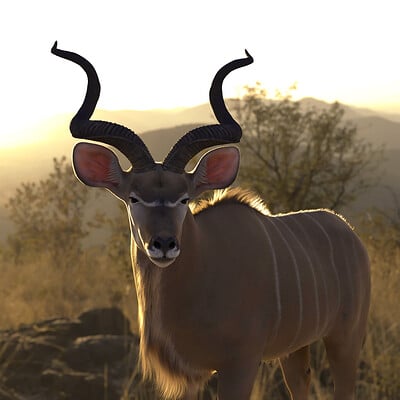An outdoor photograph captures a majestic animal, likely a greater kudu, standing on a savanna-like terrain. The kudu is mostly a light brown color with thin white vertical stripes running along its side, surpassing its front legs. The animal’s striking features include large, oval-shaped ears with pink interiors, and two prominent, thick, corkscrew-shaped, dark horns rising from its head. White markings above its dark eyes give the appearance of "angry eyebrows," as it gazes directly into the camera. The kudu also has a distinctive furry chest and a small tuft of fur on its back, which catches the warm yellow light of the early morning sun, illuminating the fine blonde hairs along its back.

In the background, the scene unfolds with beige wild grasses and sporadic trees stretching toward distant hill ranges. A mound composed of dark gray rocks is positioned to the left of the kudu, adding texture to the landscape. This captivating image, reminiscent of frames seen on Animal Planet, offers a detailed and mesmerizing view of this splendid creature in its natural habitat, ready to grace any wildlife documentary.